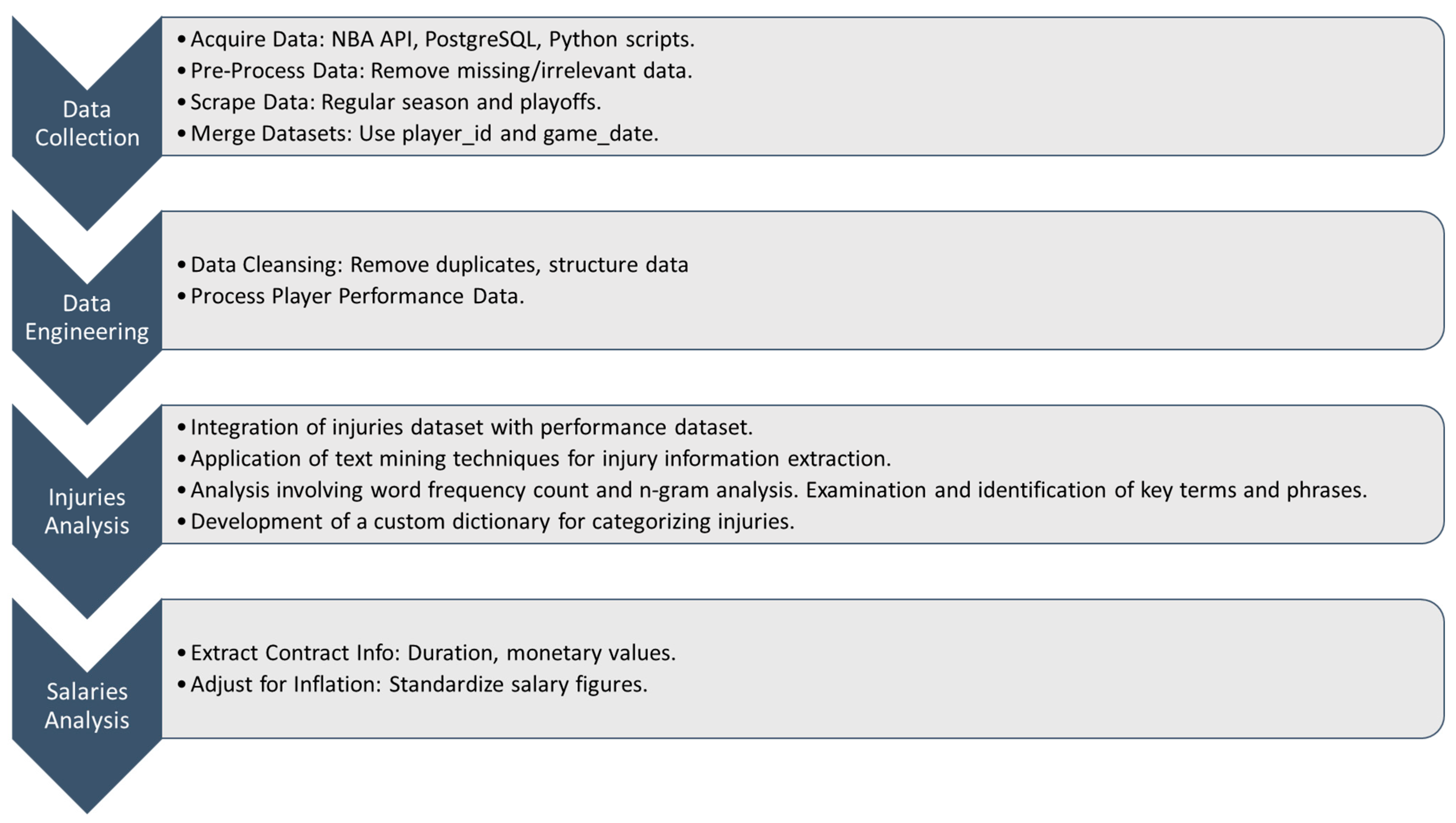The image depicts a detailed flowchart illustrating the process of data analysis in the context of NBA statistics, with four main phases: Data Collection, Data Engineering, Injuries Analysis, and Salaries Analysis. 

In the Data Collection phase, tasks include acquiring data through the NBA API, PostgreSQL, and Python scripts, followed by preprocessing to remove missing or irrelevant data. It also involves scraping data for both regular season and playoffs, and merging data sets using player IDs and game dates.

The Data Engineering phase focuses on data cleansing, which involves removing duplicate structured data and processing player performance data.

In the Injuries Analysis phase, the integration of the injuries dataset with the performance dataset is highlighted. This phase employs text mining techniques for extracting injury information, including word frequency counts and N-gram analysis, and involves the examination and identification of key terms and phrases. A custom dictionary is developed for categorizing injuries.

Finally, the Salaries Analysis phase includes extracting contract information such as duration and monetary value, adjusting for inflation, and standardizing salary figures.